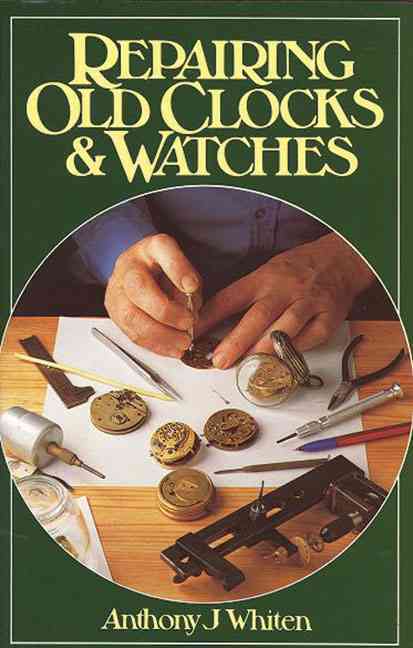This is the cover of a book titled "Repairing Old Clocks & Watches" by Anthony J. Whiten. The text, written in an old-school serif font, is displayed in pale yellow against a green background with a thin white border near the edges. At the top, the title is presented over three lines, and at the bottom, just above the white border, the author's name is highlighted. The central image, enclosed within a thin white circle, features a man's hands, partially depicting his torso clad in a blue button-down shirt. The hands are delicately working on the internal parts of a pocket watch placed on a piece of white paper positioned on a wooden table. Scattered around are various tools, including tweezers, screwdrivers, pliers, and a pencil, alongside numerous watch and clock components, indicating a meticulous repair process.